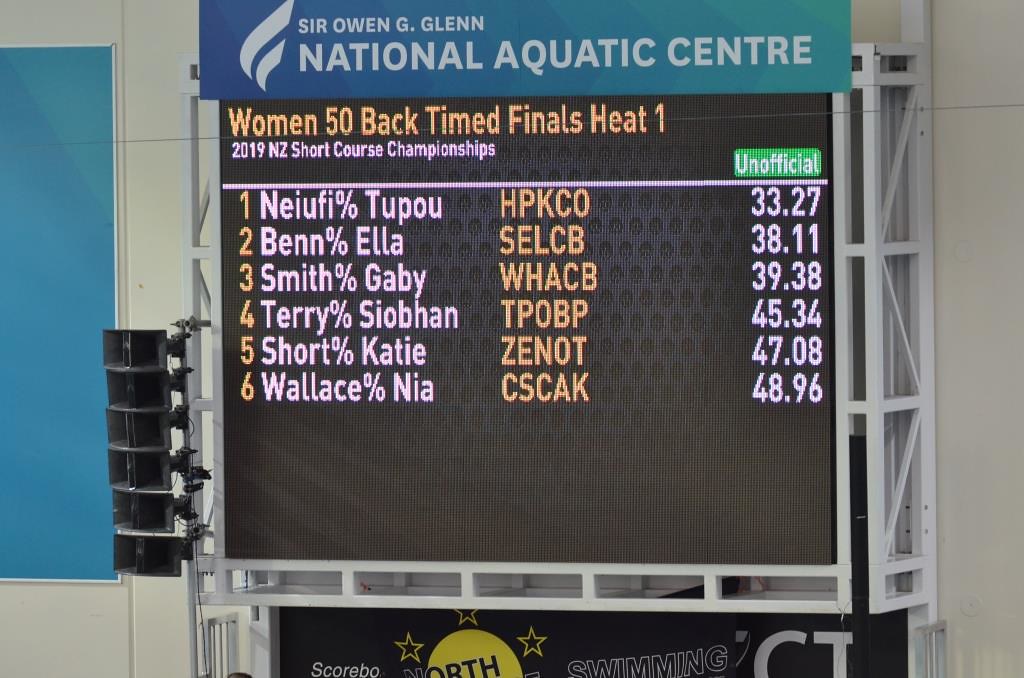The image shows an electronic scoreboard mounted on a metal frame extending from a grey-painted wall, with railings and loudspeakers on the left-hand side. At the top of the scoreboard, a non-electronic sign with a blue background reads "Sir Owen G. Glenn National Aquatic Center" in white lettering. Below this, the electronic section of the board details the event: "Women 50 Back-Timed Finals Heat 1 2019 NZ Short Course Championships" in yellow letters. The scoreboard lists six names, each accompanied by a ranking number and their respective scores. The names are displayed in an orange font, and to the right, labeled in green, are the unofficial rankings. The scores range from 33.27 to 48.96. At the bottom of the board, an advertisement adorned with yellow stars partially reads "Scorbo North Swimming CT." The scoreboard also features a raised white border around the electronic display.